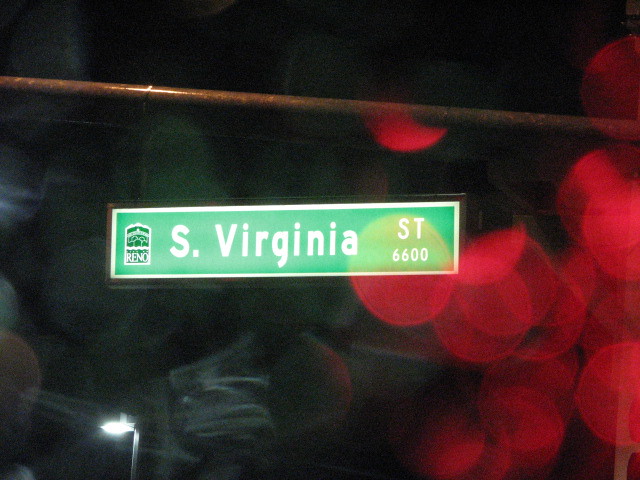This photo, taken at night from inside a car, captures a green and white street sign for South Virginia Street, specifically the 6600 block. The background is predominantly dark, with the only illumination coming from a distant street light at the bottom left corner and various red circles, likely reflections of a traffic light on a rainy window. The street sign is attached to a pole that stretches above the car. A smaller sign with the city logo of Reno appears on the left side of the main sign. An overhead wire crosses the top part of the photo, adding to the night-time ambiance. The image is blurry, giving it a smoky, unfocused effect.